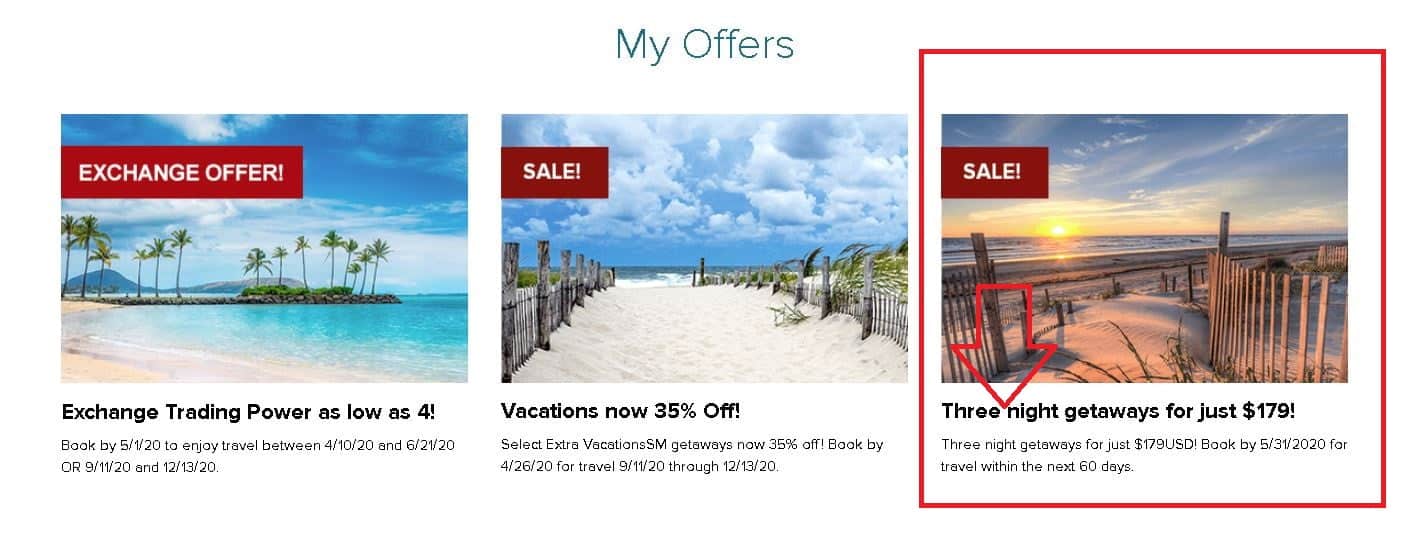This screenshot captures a section of a promotional webpage titled "My Offers" in dark teal header text. The layout features three columns, each showcasing a tropical destination with vibrant beach scenes. Each destination image is partially overlaid by a red banner with white text that originates either from the left or right side. 

- **Left Column**: The banner says "Exchange Offer." The text underneath reads, "Exchange trading power as low as 4. Book by May 1st, 2020, to enjoy travel between April 10th, 2020, and June 21st, 2020."
  
- **Center Column**: The banner here says "Sale." The text indicates, "Vacations are now 35% off," though finer details are too small to read clearly.

- **Right Column**: This image stands out with a red outlined border and arrow pointing to the offer. The banner reads "Sale." The text below details, "Three-night getaways for just $179 USD. Book by May 31st, 2020, for travel within the next 60 days."

Each image captures the allure of sunny, picturesque beachfronts, enticing viewers with the promise of tropical retreats.